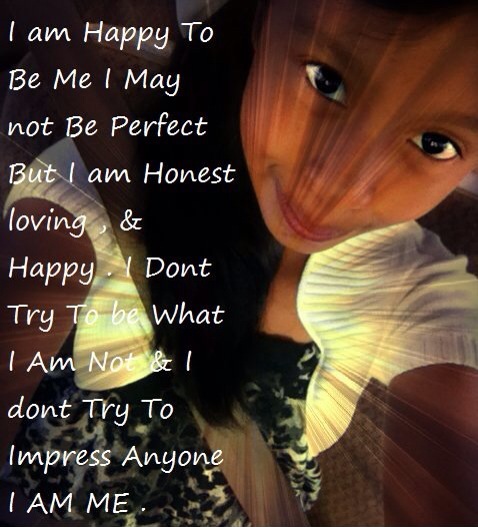The image is an inspirational quote superimposed on a picture of a young woman taking a selfie from above. She has dark skin and is dressed in a white jacket and a black floral print outfit. Sunlight casts warm shadows across her face, giving the scene a captivating and serene aura. The left half of the image features an inspiring text in white, set against the backdrop of her illuminated and contemplative expression. The quote reads: "I am happy to be me. I may not be perfect, but I am honest, loving, and happy. I don't try to be what I am not, and I don't try to impress anyone. I am me." The overall effect of the image, with its warm sunlight and thoughtful message, is both inviting and encouraging, celebrating authenticity and self-acceptance.